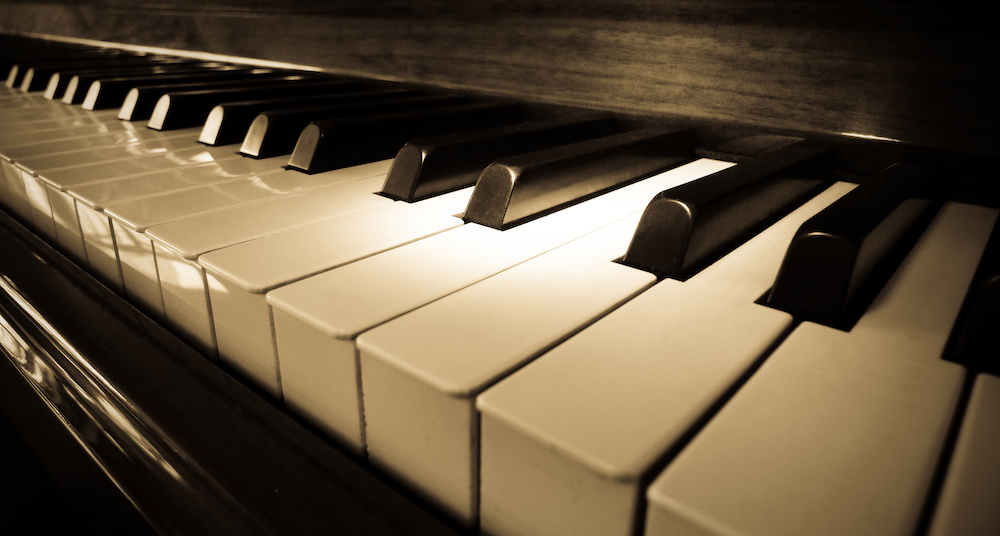This is an artistic close-up photo of a piano keyboard taken indoors from the perspective of someone standing at the right edge. The image, predominantly in black and white with a subtle yellow tint, showcases approximately 15 to 20 pristine white keys. The viewpoint creates an illusion of the keys increasing in size toward the right corner, giving a grand sense of scale. The black keys are interspersed among the white, with the top portion of the image revealing a wood grain finish of the piano, suggesting it might be composed of a dark, glossy wood. The keys have a reflective sheen, particularly noticeable on the polished black surface at the bottom and a reflective spot near the center-right. The absence of text ensures focus on the intricate details, from the clean keys to the grain of the wood, highlighting the fine craftsmanship of the instrument.